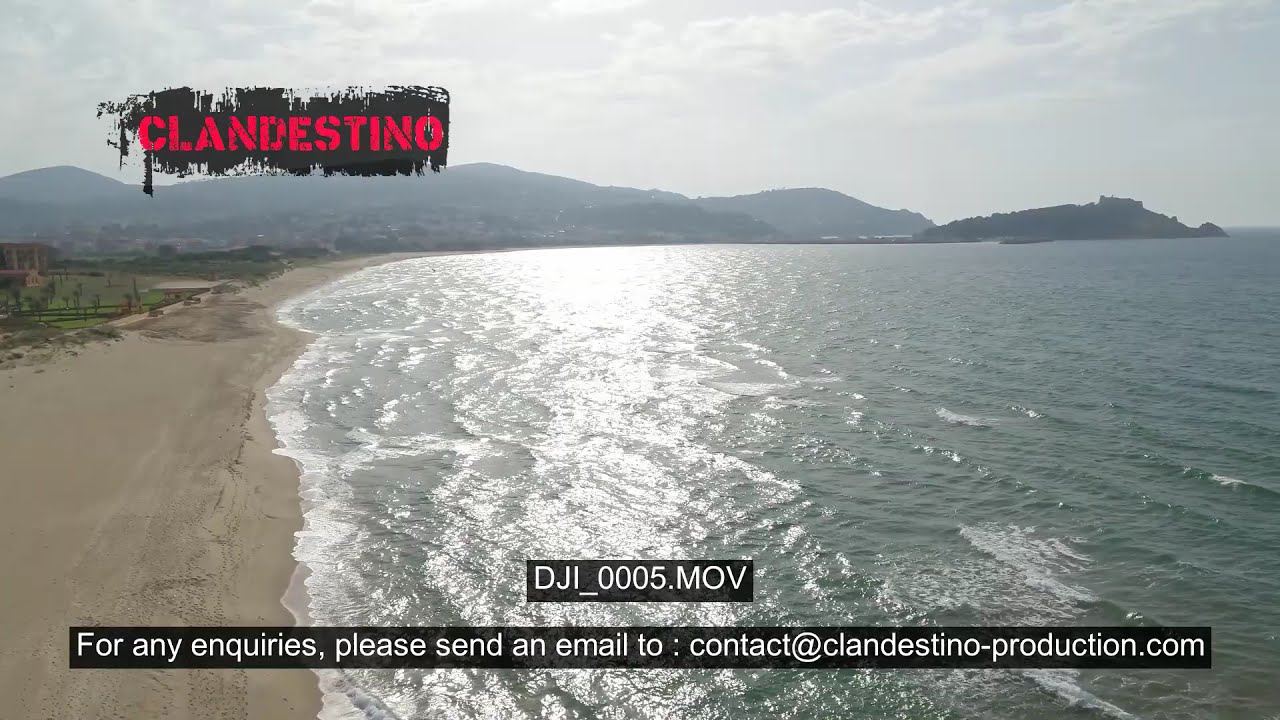This image portrays a serene beach scene with soft, sandy shores and gently reflecting, slightly choppy waters suggesting a breeze. The horizon is adorned with hazy mountains and hills in varying shades of gray and black, with hints of green vegetation peeking through. Clouds diffuse the light, adding to the tranquil ambiance. In the top left corner, the word "CLANDESTINO" in red uppercase letters stands out against a black graffiti-like background, possibly indicating the beach's name. At the image's bottom, a black banner displays "DJI_0005.MOV" in white text, signifying the file name, followed by a contact prompt: "For any inquiries please send an email to contact@clandestinoproduction.com." This indicates that the image is part of a video likely produced by Clandestino Production.